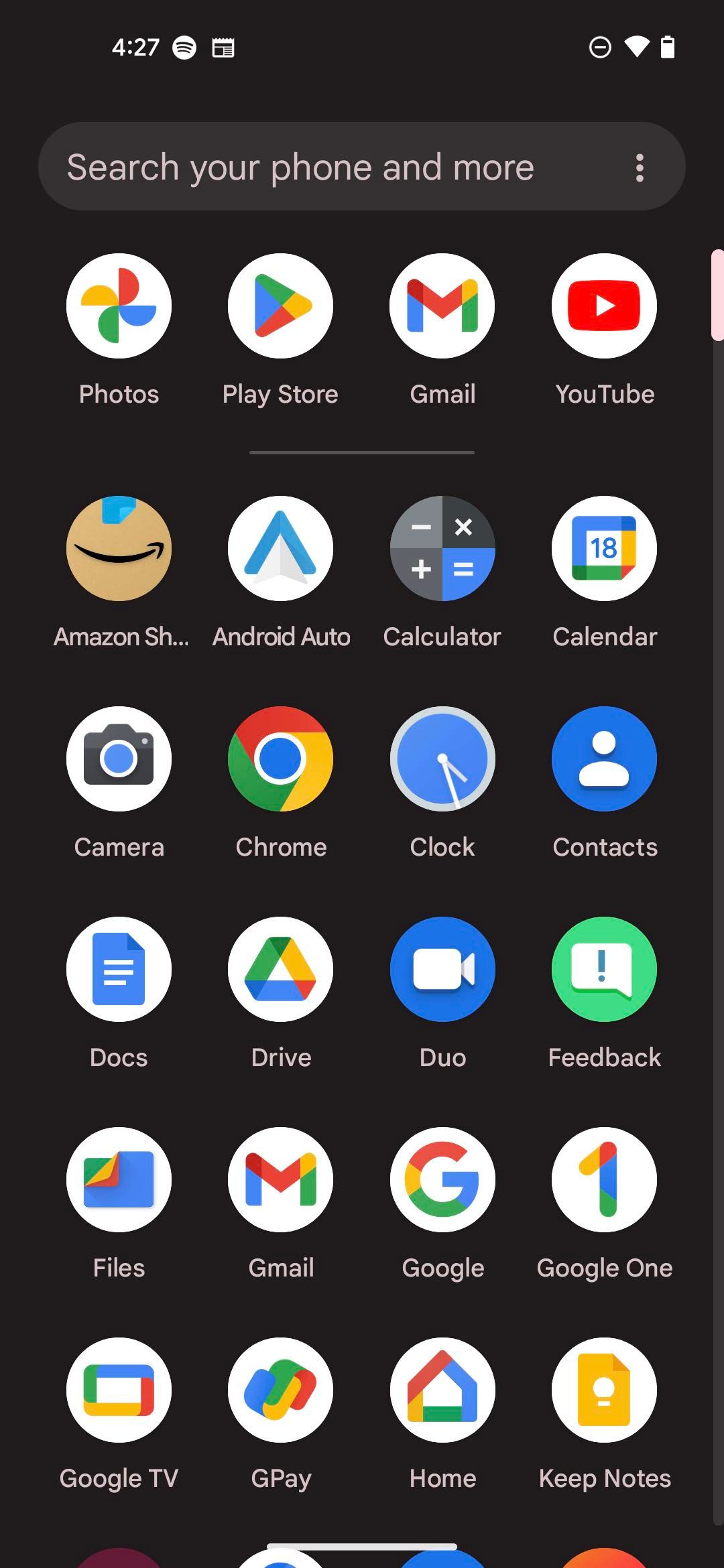A screenshot of an Android smartphone's home screen showcases a range of application icons neatly organized in a grid. At the top left, the current time is displayed, while the top right corner indicates the battery status. Dominating the upper section is a gray search bar with the text "Search your phone and more." Directly below the search bar, several app icons are prominently visible: Photos, Play Store (illustrated by a pinwheel), Gmail, YouTube, and Amazon Shopping, which is partially cut off. Additional apps like Android Auto, Calculator, Calendar, Camera, Chrome, Contacts, Docs, Drive, Duo, Feedback, Files, Gmail, Google, Google One, Google TV, GPay, Home, and Keep Notes form the visible part of the list. A scrolling bar on the right side suggests that there are many more icons below the current view. Notable icons include the brown Amazon Shopping icon with an arrow, the colorful Chrome icon, the Camera icon, and the Calculator icon. The overall impression is of a well-organized digital toolset, ready for various tasks and activities.